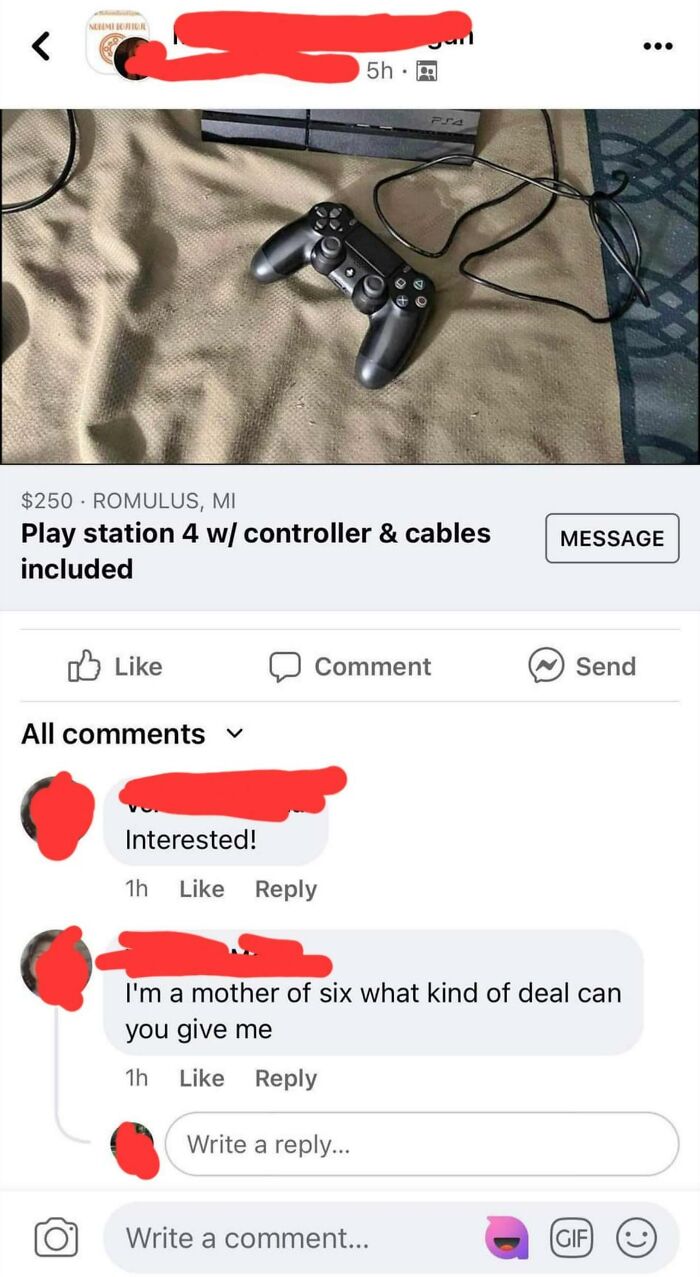This is a detailed screenshot from a sales advertisement, featuring a PlayStation 4 set for sale on a white background. The main image occupies the upper portion, showing a black game controller placed in front of a partially visible PS4 console. Both items rest on a bed layered with a tan blanket over a blue one. Below this, a light gray rectangular section displays vital information, starting with the price of $250 and the location noted as Romulus, Michigan. The text "PlayStation 4 with controller and cables included" provides a brief description of the offer.

On the right side of this gray box, there is a dark gray rectangular button labeled "Message" in black text. Beneath this, typical Facebook interaction icons are lined up: a "like" button with a thumbs-up icon, a "comment" button with a speech bubble icon, and a "send" button marked by a speech bubble containing a lightning bolt. Below these buttons, the section for comments starts with "All Comments" in black text. Several user comments are visible, accompanied by circular profile pictures that have been blurred out with red marker, and names that have been erased. Example comments include statements such as "Interested" and "I'm a mother of six. What kind of deal can you give me? Thank you." The title of the item, positioned at the top of the screenshot, has been obscured.